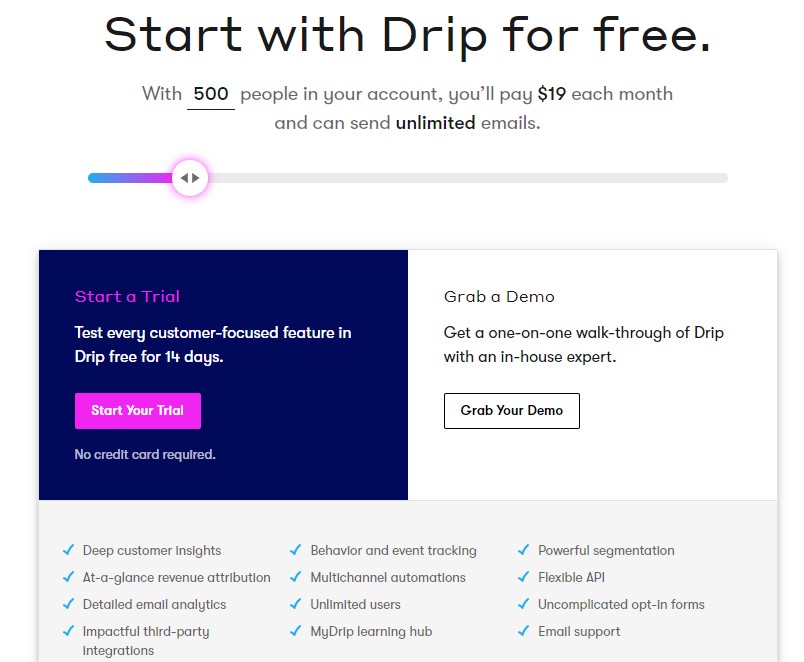The image features a clean white background with prominently displayed text and various design elements. At the top, there's a headline reading "Start with Drip for Free," followed by text stating, "With 500 people in your account, you'll pay $19 each month and can send unlimited emails." This line is underlined for emphasis. 

Below the main text, there's a visually attractive horizontal gradient line transitioning from blue to purple. In the middle of the image, there's a circular icon featuring left and right arrows.

Dominating the center is a large blue box that encapsulates a smaller, very dark blue box. Inside this dark blue box, the text reads, "Start a trial. Test every customer-focused feature in Drip free for 14 days." Directly below this, a small purple button invites action with the words, "Start Your Trial. No Credit Card Required."

On the right side of the image, there is a segment with a white background. It contains a heading that says, "Grab a Demo." Beneath this, it reads, "Get a one-on-one walkthrough of Drip with an in-house expert." Below these lines, there's a button labeled, "Grab Your Demo."

The bottom section of the image is filled with various detailed feature highlights on a blue background. Each feature is accompanied by a blue checkmark and includes: 
1. Deep customer insights at a glance, 
2. Revenue attribution, 
3. Detailed emoji analytics, 
4. Impactful third-party integrations,
5. Behavior and event tracking,
6. Multi-channel automations,
7. Unlimited users,
8. My Drip learning hub,
9. Powerful segmentation, 
10. Flexible API,
11. Uncomplicated opt-in forms,
12. Email support.

This detailed layout effectively showcases Drip's offer and its robust set of features in an organized and visually appealing manner.